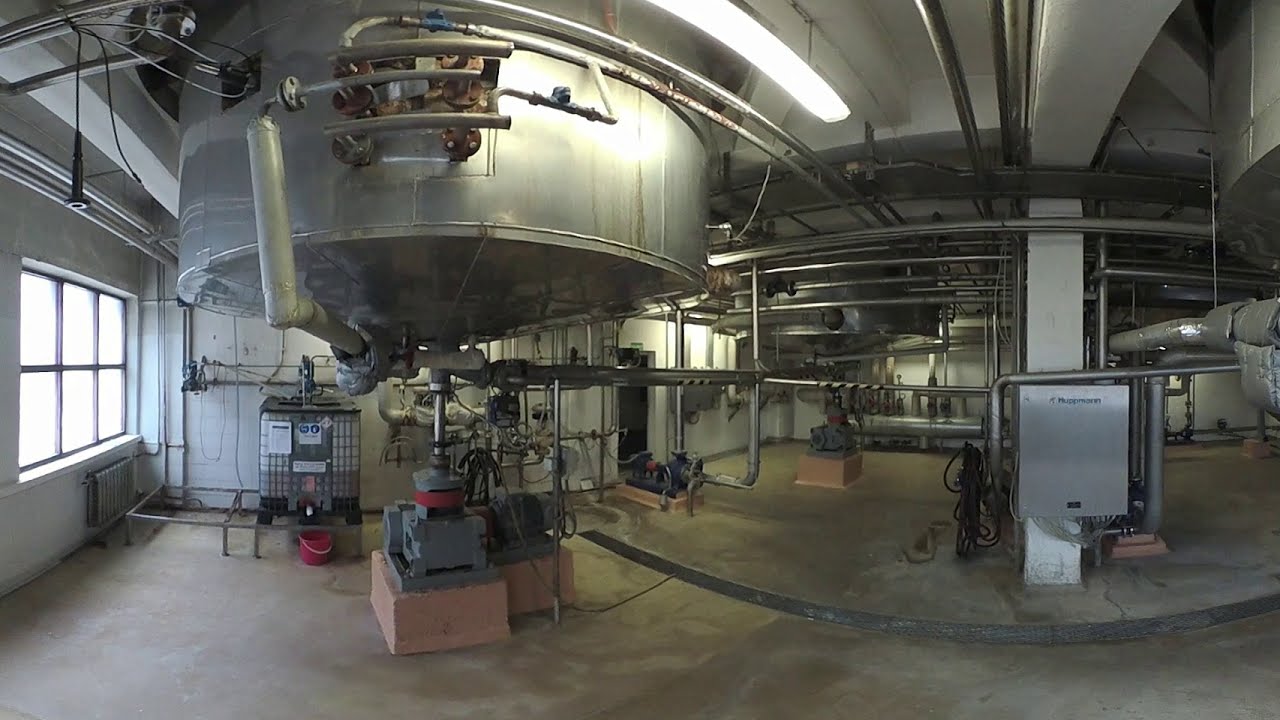The image depicts a clean, industrial scene within a large warehouse-like setting, likely a manufacturing or processing plant. The concrete floor supports a variety of stainless steel and metal equipment, characterized by an intricate network of piping and tubing. Central to the image is a large, silver-colored holding tank elevated above the ground, featuring a pipe connected to what appears to be an electric pump mechanism at the bottom. Adjacent to this tank, there is a red bucket. 

To the left, a wall with windows allows light to filter into the space, highlighting additional details such as a heater radiator near the windows and a fluorescent light fixture affixed to the ceiling, illuminating the area around the tank. Three horizontal pipes extend from the top of a chemical vat positioned to the left, suggesting robust chemical processing capabilities. The right side of the image reveals more complex piping and machinery, evoking a boiler room setting. The presence of the words "H-U-P-P-R-N-P-R-I-N," though not entirely clear, suggests some form of labeling or branding within the plant. Despite the industrial nature of the scene, the area appears well-maintained and tidy.